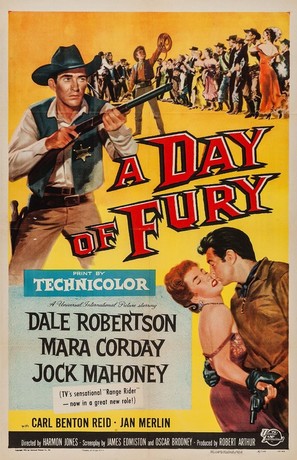This is an old-school, Western-style movie poster with a yellowish-orange background. The main title, "A Day of Fury," is prominently displayed in red, spiky, almost edgy font with a black shadow and white trim. The bottom left corner features a teal box that announces "Print by Technicolor," with some undecipherable cursive text in pale blue beneath it. Key actors' names—Dale Robertson, Mara Corday, Jock Mahoney, Carl Benton Reid, and Jan Merlin—are listed across the poster in various places. A white box partially overlaps the pale blue writing, bearing the text "TV Sensation, Range Rider," indicating a connection to the well-known television series. 

Visually, the poster includes central imagery of a cowboy with a sheriff's badge holding a rifle. Some townspeople are depicted towards the top, and towards the bottom, a man dressed in a brown shirt embraces and kisses a woman with red hair who is wearing a dark red dress. The sheriff is characterized in a green vest, brown pants, and a black cowboy hat, adding a distinctive flair to the vintage aesthetics of the poster.